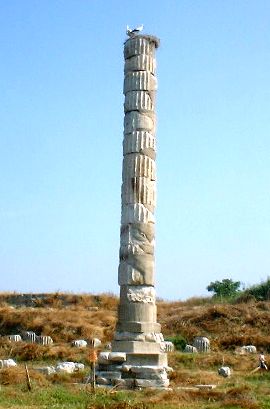This full-color outdoor photograph taken in bright daylight features a striking scene under a clear, cloudless blue sky, with the majority of the image showcasing this expansive sky. In the foreground stands a tall, ancient stone pillar, likely made of gray marble or limestone and reminiscent of historical sites found in places like Greece or Rome. The pillar, though in a state of significant disrepair, stands resiliently at an estimated height of around 30 feet. Its construction appears mismatched, composed of stacked circular segments that don't perfectly align, giving it an almost patchwork appearance. The square base of the pillar contrasts with the circular segments above. At the pinnacle of this weathered column rest two birds, adding a touch of life to the scene.

The area surrounding the tall pillar is scattered with numerous small, broken-down pillars and segments of similar material, akin to rubble from a previously toppled tower. These fragments suggest a once grander structure now reduced to ruins. The ground is covered with patches of green grass interspersed with brown scrub, contributing to the scene's rugged, natural beauty. Encircling the base of the tall pillar is a staked-off area, likely intended to prevent further human interference and preserve what remains of this historical relic.